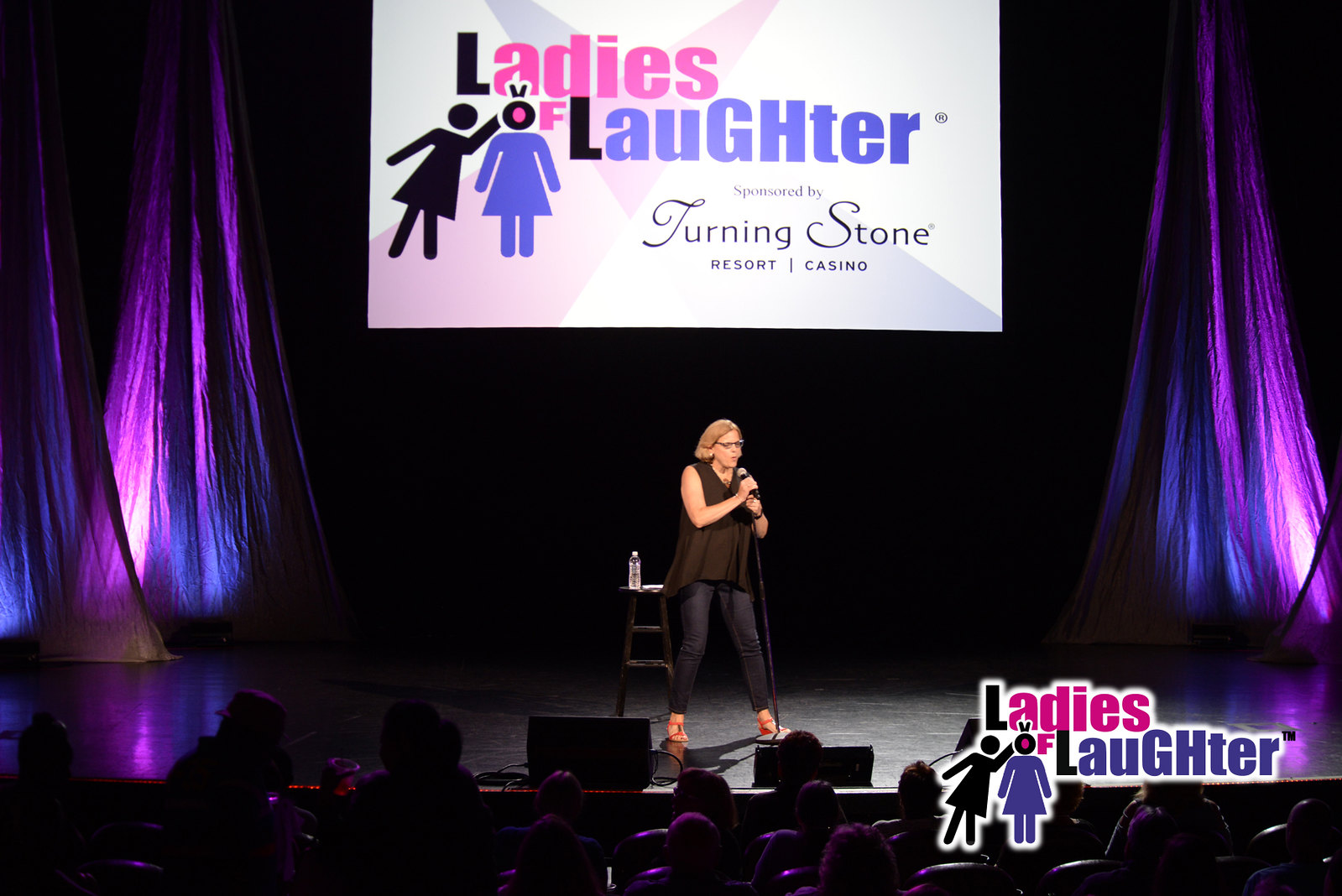In the image, a lady stands on a black stage, performing at an event called "Ladies of Laughter," sponsored by Turning Stone Resort Casino. She has short blonde straight hair and wears glasses, a brown sleeveless v-neck shirt, and tight denim jeans, accented by red heeled shoes. Her hands are wrapped around a microphone as she speaks to the audience.

Behind her is a wooden stool with a bottle of water on it, possibly holding a piece of paper as well. The backdrop features a large banner with the event's name and two symbolic outlines of women wearing dresses, reminiscent of women's restroom signs. One figure is in black, giving bunny ears to the other figure in pink or purple.

The stage is surrounded by purple drapes on either side, adding to the vivid ambiance. The audience, visible from the back with some members holding drinks, attentively watches the performance. In the bottom right corner of the image, the "Ladies of Laughter" logo reappears, consistent with the banner above the performer.